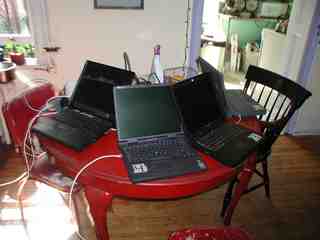The image is a grainy, low-resolution photograph of what appears to be a room in a house, likely a dining room or kitchen area. At the center of the room stands a circular wooden table painted red. On the table, there are four black laptops arranged in a semicircle, all open with their screens turned off. The laptops vary slightly in design, with some featuring different-colored buttons and logos positioned inconsistently, suggesting they are older models from around the mid-2000s. Each laptop is connected to white charging cables running to the sides.

A black dining chair is pulled up to the right-hand side of the table. Another chair, possibly more modern with metal and upholstery, is situated on the left side of the table. In the background, the upper right-hand corner reveals an open doorway leading to another room, which might be a kitchen. The doorway frame is colored purple. Additionally, the room has a wooden floor of a darker tone, and a window is partially visible in the upper left-hand corner of the image, with some greenery, possibly plant pots, placed on the windowsill. Near the window, there is another table with a few items on it, including a silver pot and a white bottle. Overall, the photo depicts a cluttered yet functional space with a nostalgic touch.